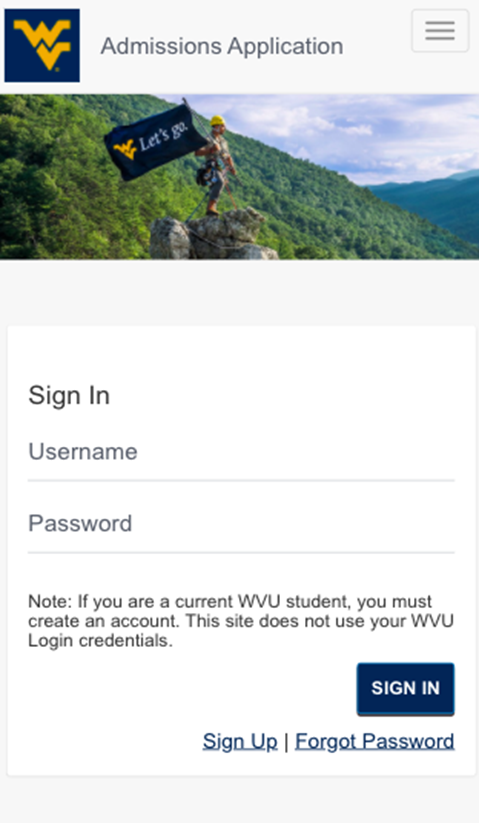The image features a gray background at the top, transitioning into the interior view dominated by a navy blue box. This box prominently displays the letters "WF," which likely stand for West Virginia University. Adjacent to these letters, in black text, are the words "Admissions Application." Below this, there's a gray box outlined in a darker gray, containing three gray lines and an image of a person standing on a large gray rock next to a green mountain. Above the rock are yellow clouds, and the individual is holding a flag that says "Let's Go!"—the flag shares the same color scheme as the previously mentioned boxes with "WV" in yellow.

In this gray space, a white box is present, featuring sign-in fields on the left-hand side. In black text, it first states "Sign-In," followed by fields labeled "Username" and "Password," each with a thin gray line underneath for users to type in their credentials. Beneath the password field, black text states: 
"Note: If you are a current WVU student, you must create an account.
This site does not use your WVU login credentials."

At the bottom of the white box, a button reading "Sign-In" in white text stands out against a navy blue rectangle. Below this, in navy blue text, the options "Sign Up" and "Forgot Password" are visible.